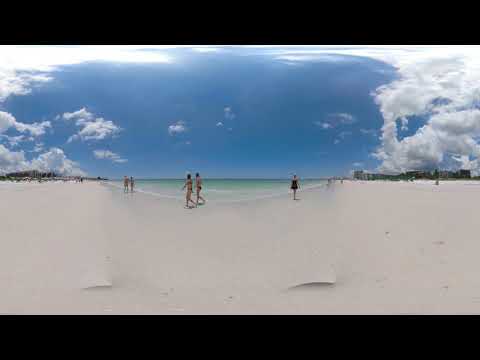This panoramic photograph captures a serene beach scene on a bright, sunny day. The composition is divided into two halves: the upper half showcases a vivid blue sky adorned with billowy clouds that frame the left, right, and top perimeters, while the bottom half features a peaceful sandy beach and a sliver of the greenish ocean. In the center of the image, two women in bikinis walk to the left, while a couple strolls along the left side and a singular woman in a black bathing suit is seen on the right. The sand remains undisturbed, appearing perfectly flat without any visible footprints. On either end of the horizon, where the sky meets the shore, patchy shrubs or green grass and some indistinct land features can be observed. The image is bordered by black rectangular strips on the top and bottom, further framing this tranquil coastal moment.